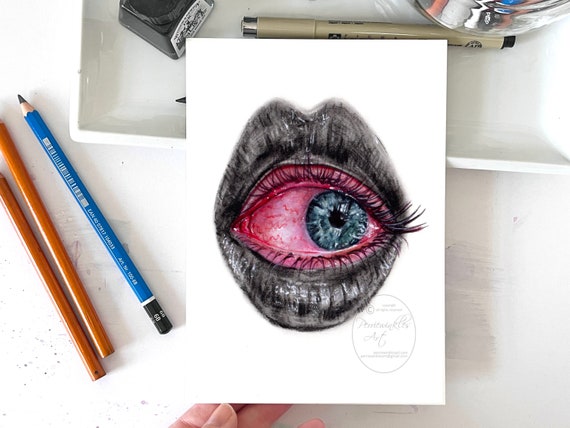The image captures a detailed photograph of a pencil drawing enhanced with colored pencil and pen, possibly including ink, creating a surreal composition. The drawing is on white paper and prominently features a black and gray shaded set of lips with a striking red eyeball positioned between them. The eye is distinctly bloodshot and exhibits long, detailed eyelashes. Its iris is a captivating mix of blue shades, suggesting a look of fear. The photo is taken in what appears to be an artist's studio, as indicated by various art supplies around the drawing. Three pencils—one black and two yellow—lie to the left, and a fine-point pen is positioned horizontally at the top. An inkwell is also displayed nearby. The drawing itself seems to be held up by a hand with polished nails, partially visible at the bottom of the image. Text at the bottom of the drawing blends faintly with the white paper, making it difficult to discern.